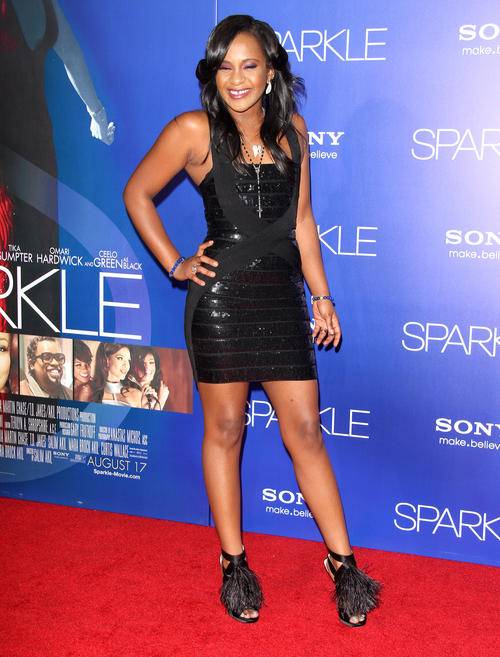This is a detailed color photograph of Bobbi Kristina Brown posing on the red carpet at the premiere of "Sparkle," a movie associated with her mother, Whitney Houston. The backdrop is a blue canvas adorned with the words "SPARKLE" and the Sony "make.believe" logos in white print. To the left, part of the movie poster is visible, featuring images from the film, including a man with glasses and a beard, and three women clustered together.

Bobbi Kristina is wearing a sleeveless, skintight black leather mini dress with a silver zipper running down to her waist. The dress has shiny, horizontal bands and an incorporated off-black shoulder strap. She accessorizes with a black rosary-style necklace with a cross that hangs near her waist, large white earrings, and bracelets on both wrists. Her black strappy sandals feature fringes reminiscent of fur balls, and she has a ring on her finger. Bobbi's makeup includes purple eyeshadow, and she has long black hair.

She stands confidently on the red carpet, smiling with a visible gap between her teeth. Her eyes appear closed in the image, adding a serene touch to her joyful expression.